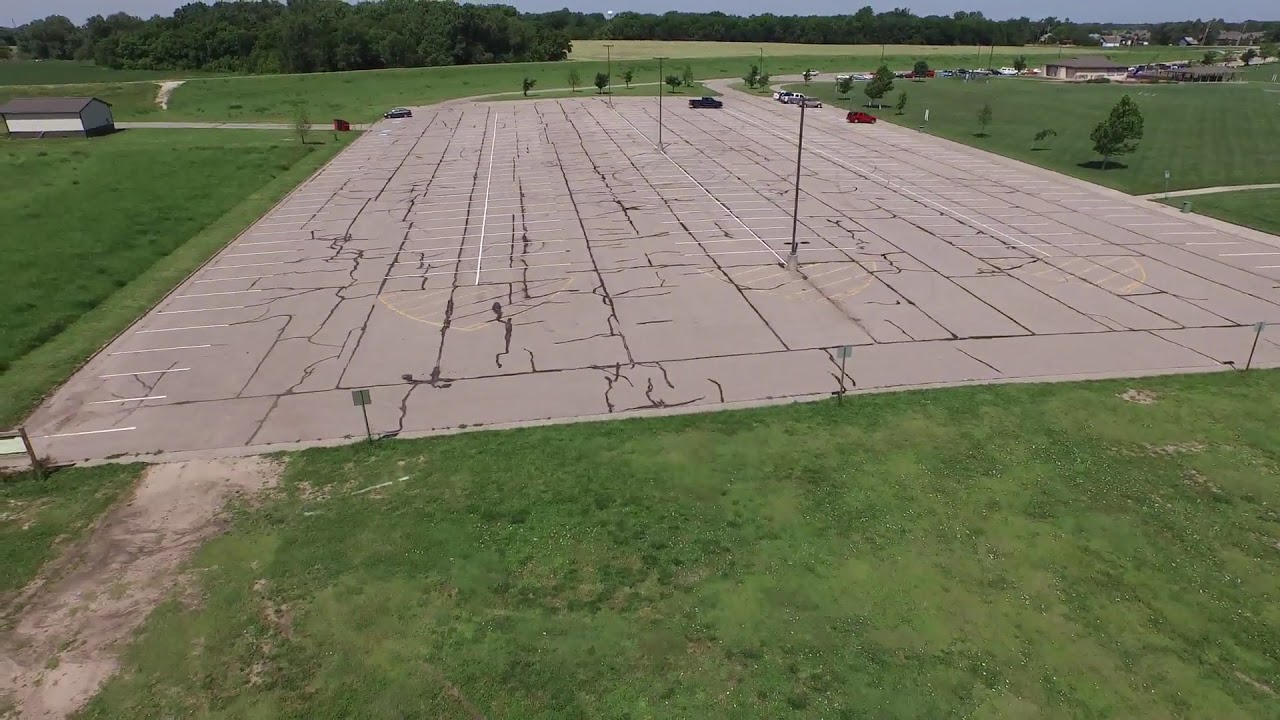This outdoor daytime photograph captures a nearly empty, large cracked parking lot, predominantly light grey with numerous dark patches and white parking space lines. A series of black light poles lines the center. In the foreground, lush green grass borders the lot on all sides, with more grass stretching out to the left and right. On the left side, a small, long, white building sits on the grass. To the right, beyond more grass, lies another small building with an adjacent driveway or parking area filled with multiple cars. In the parking lot itself, a dark-colored car is parked on the far-left side, while a cluster of five or six vehicles, including a black truck, a red SUV, a silver car, and a white pickup, are positioned on the far-right. Surrounding the entire scene are expanses of grass fields, hills, trees, and a few residential buildings scattered in the backdrop, giving the impression of a quiet, suburban setting.